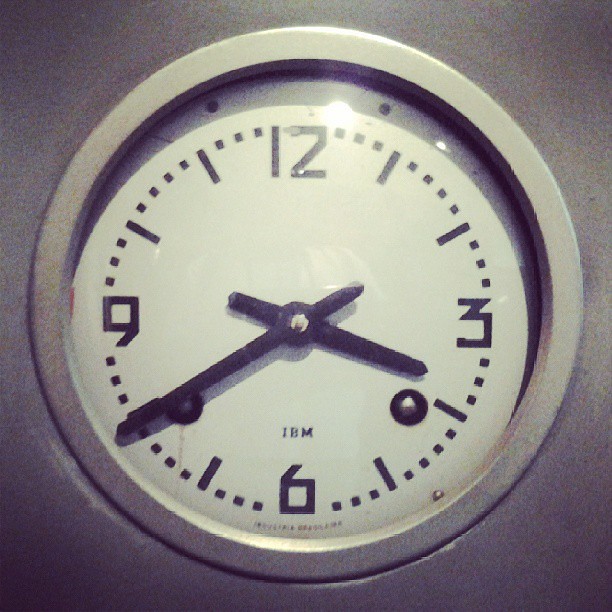This image features a distinctive metal clock with a sunken white face that appears to have slightly detached from its proper position, resting lower within the clock’s frame. The clock's face is adorned with black numbers and hands, with the numerals having a notably boxy appearance, particularly the 6 and 9, which gives the clock a unique aesthetic. To the left side of the clock, there is a noticeable scrape in the metal, revealing red undertones beneath the gray exterior. Additionally, the clock has two bullet holes, suggesting that it might be designed to be wound up through these apertures. The overall design combines utilitarian and industrial elements, characterized by its visible wear and distinct numbering style.